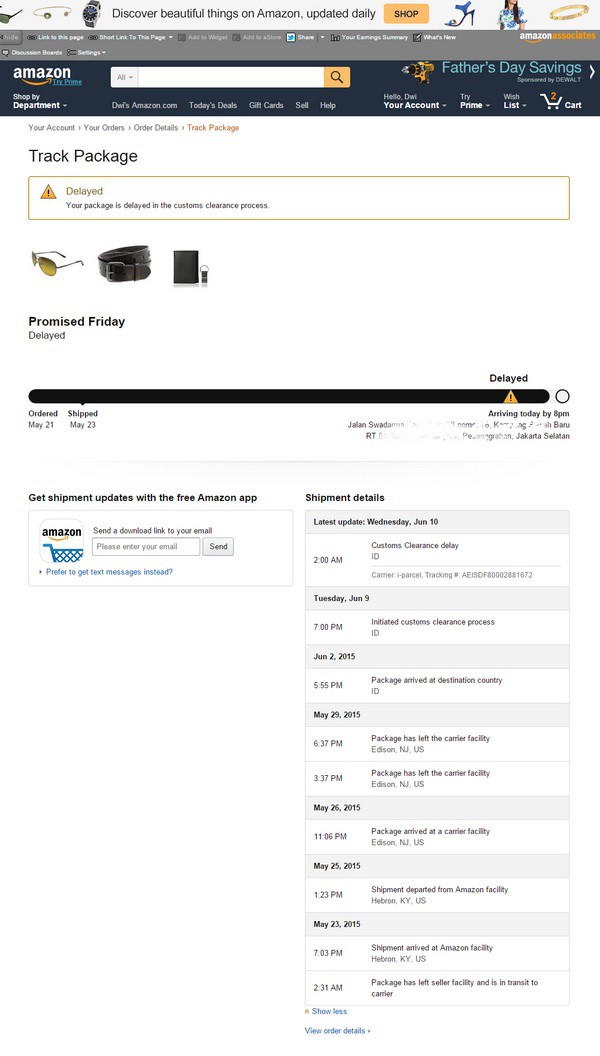Screenshot of the Amazon website:

At the top of the screen, there's a white banner that reads, "Discover beautiful things on Amazon, updated daily" with a yellow "Shop" button to the right. Below this, there's a gray banner featuring links, though the text is too small to discern. Subsequently, a navy blue banner appears with the Amazon logo on the left and a search field with a yellow magnifying glass button on the right. In light blue font to the right of the search field, it says "Father's Day savings."

Further down, a white menu bar displays options such as "Departments," "Your Account," "Wish List," and "Cart" in black font. Beneath this, there is a yellow triangle with a black exclamation point, indicating an alert. The message inside the yellow border states, "Your package is delayed."

Below the alert, three images are displayed, including a photograph of sunglasses and two other indistinguishable items. Below these images, it says, "Promised Friday," followed by "Delayed."

Next, a navy blue progress bar featuring different dates is visible. It includes another yellow triangle with an exclamation point and the word "Delayed."

At the bottom, there's a section promoting shipment updates through the Amazon app with a field to enter information and a "Send" button. To the right, shipping details are provided with various times and shipment updates.